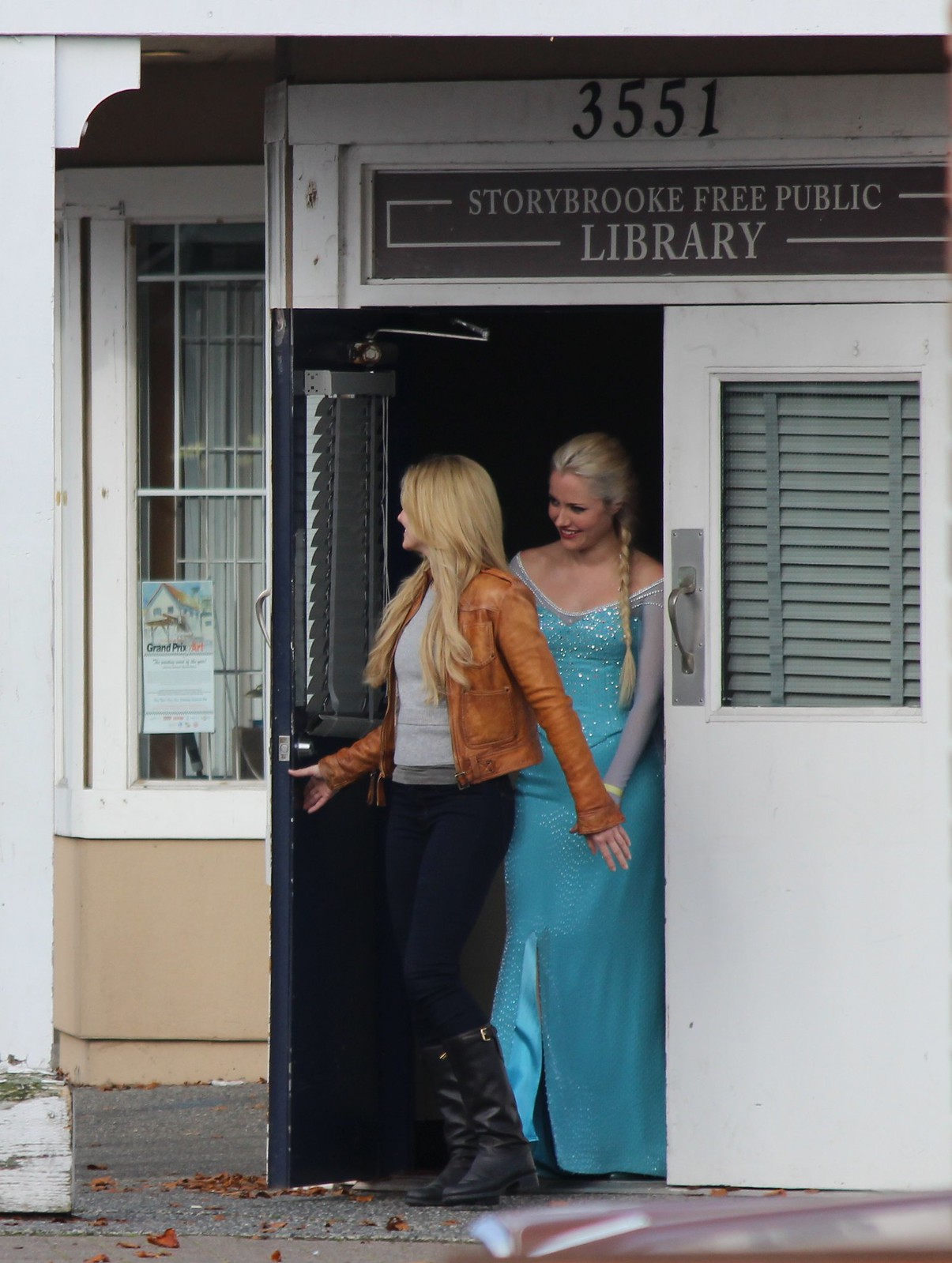In this image, two blonde women are exiting the Storybrooke Free Public Library through a set of double swinging doors. Above the doors, there is a sign indicating the library's name along with the address "3551." 

The woman in the foreground is pushing the door open; she has long blonde hair cascading down to her stomach, partially obscuring her side profile. She is dressed in a brown leather jacket over a gray shirt, paired with black pants, and black boots. Her ear is barely visible due to her hair covering it.

Trailing behind her is another blonde woman, dressed in a floor-length, teal blue dress that resembles Cinderella's style. The dress has a sparkly bodice, and her hair is styled in a braid pulled behind her. 

The library appears aged, noticeable by the weathered wooden post next to the door. The door, with a white exterior and a dark-colored interior, also has blinds over the windows. To the right of the door, a brown concrete wall and a window showing a small picture of a house can be seen. Both women are stepping out onto the sidewalk, with daylight illuminating the scene.